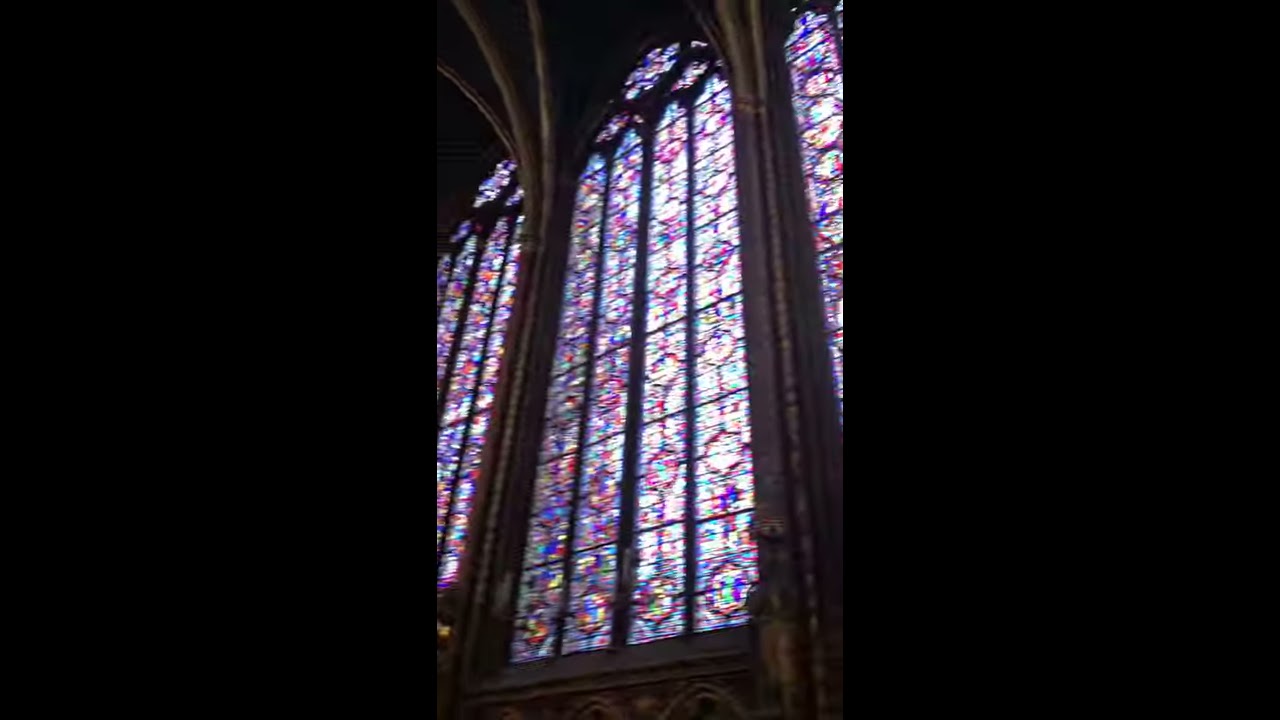This image captures the interior of a church, showcasing three towering stained glass windows that dominate the scene. The windows are anchored by large, white stone pillars that feature ornate carvings and arch gracefully towards the top, framing the colorful glass. Each stained glass window is characterized by its tall, rectangular shape, rounded at the top like a bullet. The windows are segmented into rectangular panels, with four panels per row and six rows that ascend to the rounded top, culminating in elaborately curved sections.

The stained glass itself is a mosaic of vibrant colors—reds, blues, greens, purples, and pinks—arranged in intricate designs, including octagonal patterns in the center of each panel. The sunlight streaming through these ornate windows bathes the interior in a kaleidoscope of hues, enhancing the majestic and serene atmosphere of the space.